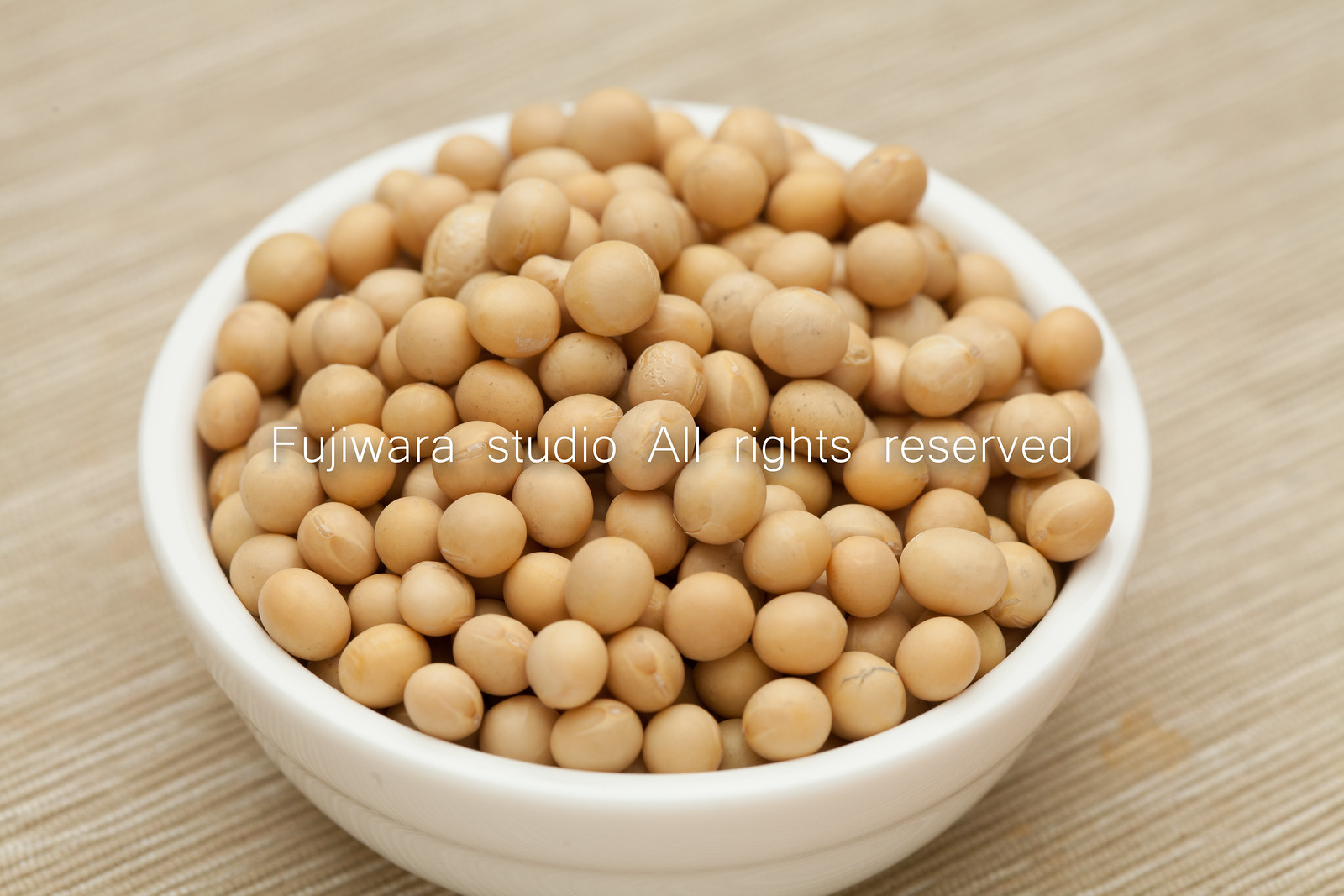This image features a close-up of a small, round white porcelain bowl filled with light beige soybeans. The bowl, with its distinctive lips that slightly indents toward the base, is set on a textured, straw-like placemat with diagonal, parallel lines in light beige and white. The soybeans are smooth, uniformly round, and slightly piled above the rim of the bowl, resembling peas. Prominently displayed in white text across the center of the image are the words "Fujiwara Studio. All rights reserved."